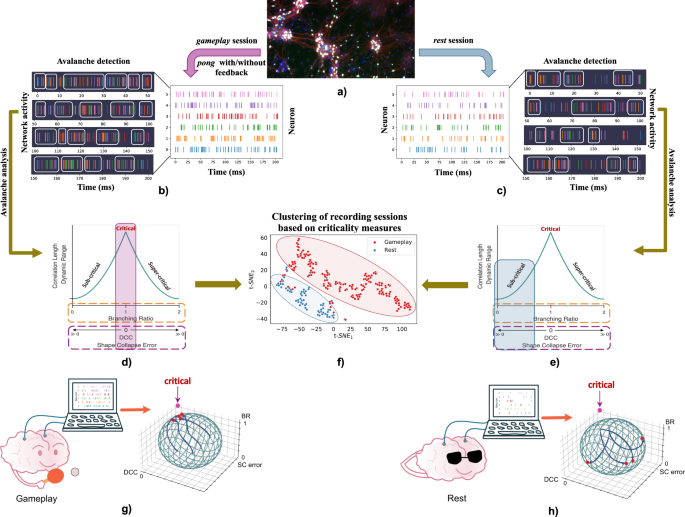The image presents a complex scientific diagram set against a white background, focused on the "clustering of recording sessions based on criticality measures" displayed centrally. At the top center, Section A features a galaxy-like, black theme with neuron-like connections, indicating an extensive network. The upper part includes labels such as "gameplay session: Pong with and without feedback," "avalanche detection," and "avalanche analysis." There are various arrows and labels, including a purple arrow pointing downwards and a blue arrow to the right labeled "rest session." 

The left side highlights the term "avalanche detection" alongside neuron time-related graphics and golden arrows pointing towards bar graphs labeled "branching ratio critical," which parallel similar structures on the right side. The central focus, F, encapsulates the criticality clustering, involving red and blue dot clusters indicative of statistically significant data points. The bottom section, G and H, illustrates a brain connected to a computer, depicting connections to an XYZ 3D brain mapping system. Overall, the image comprises 10 interconnected graphs with intricate arrows and explanations, reflecting detailed analysis on recording sessions and their criticality measures, encapsulated with scientific themes throughout.